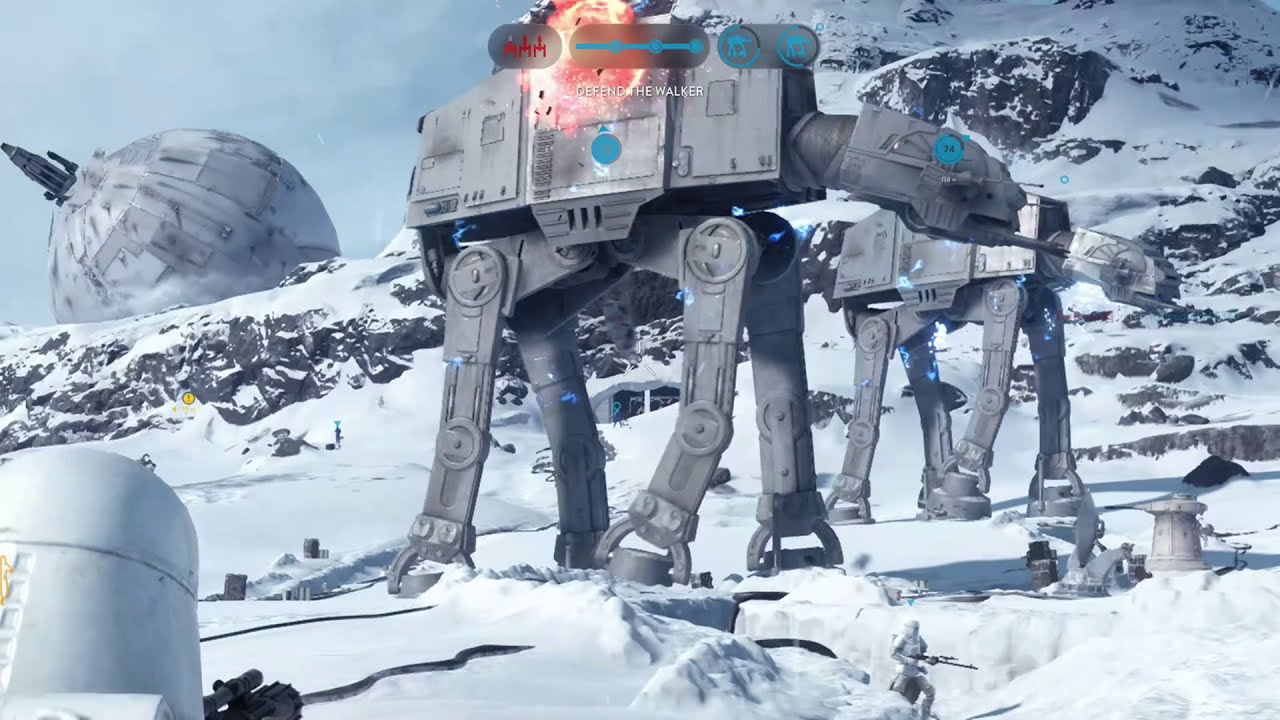The image showcases a dramatic screenshot from a Star Wars video game. Dominating the scene are two large, four-legged war machines known as "walkers," with one prominently centered and another slightly behind and to the right. The backdrop reveals a snow-covered mountainous landscape, casting a stark contrast with the battle in the foreground. The primary colors in the scene include various shades of gray from the armored machines and figures, bright splashes of red and yellow indicating fire and damage, and touches of aqua blue likely representing health levels or other game indicators. The text "Defend the Walker" is prominently displayed at the top of the screen. Additional elements include a large spherical object to the left, a storage unit in the bottom left corner, and a small figurine fighter with a gun positioned near the main walker. The overall scene suggests an intense moment of defense in an outdoor, snowy battleground, encapsulating the high-stakes action typical of a Star Wars conflict.